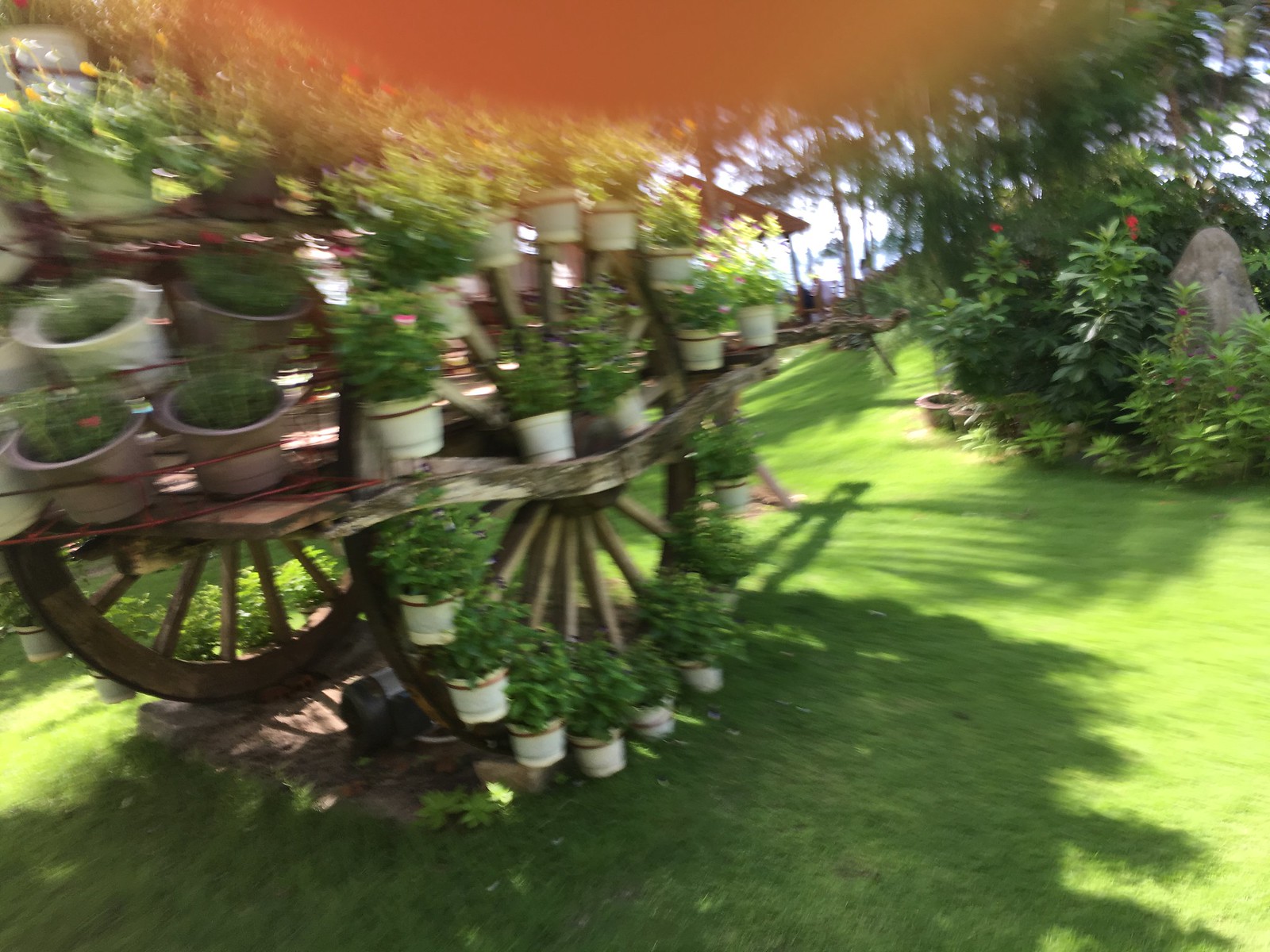The image showcases a somewhat blurry landscape-style photograph of a charming and decorative garden scene. Despite the photographer's thumb partially obstructing the top portion of the frame, the vibrant details of an outdoor setting can still be discerned. The garden features a well-maintained expanse of green grass that gently slopes upwards on the left side. A path forks in the center of the scene, with the right side of the fork revealing a rich patch of greenery. This area includes a diverse collection of plants, trees, a large rock, and a patch of exposed soil, suggesting that the path curves around this natural divider. On the left side of the path, a whimsical wheeled structure adorned with potted plants enhances the garden's decorative appeal. The scene captures the serenity and careful design of an ornate outdoor landscape.